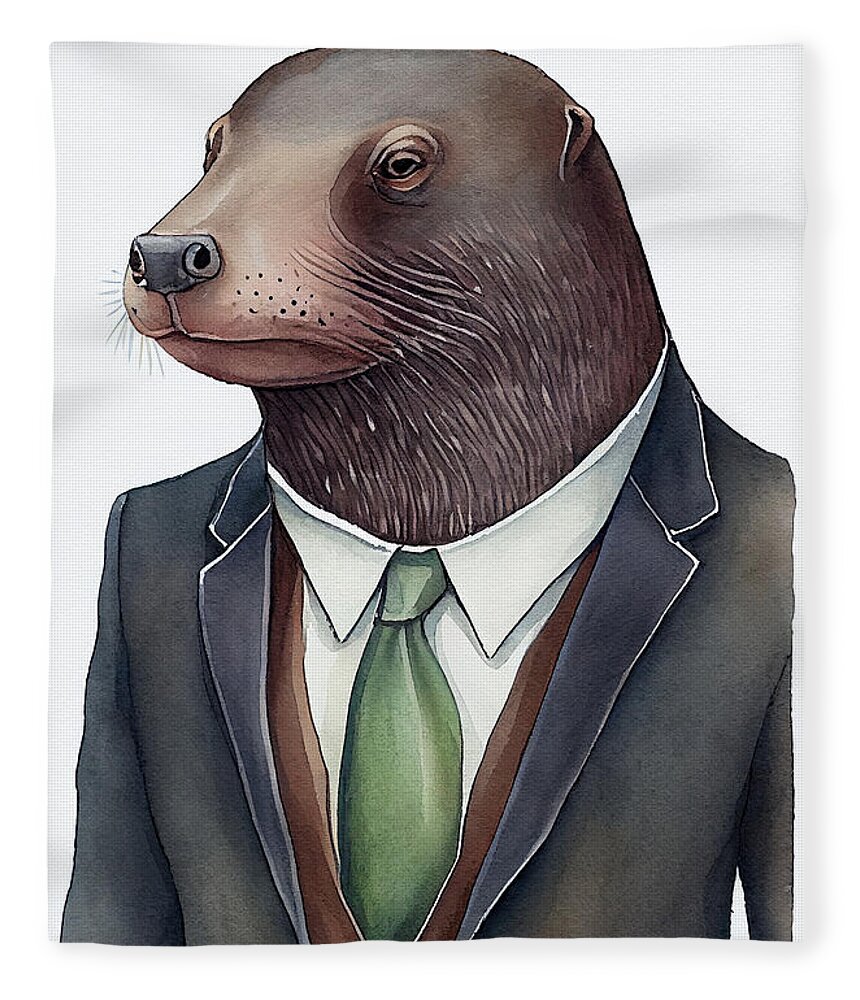This is a detailed watercolor painting set on a textured white background, depicting a unique anthropomorphic figure. The body is that of a man adorned in formal attire, which consists of a blue suit jacket over a white dress shirt, complemented by a green tie and a brown vest. The figure's head, however, is that of a walrus, characterized by its brown color, rounded small eyes, and a black nose. Distinctive whiskers extend down both sides of the face and neck, with fine lines of white fur scattered throughout the brown fur. The walrus head appears solemn and somewhat indifferent, capturing the stoic demeanor typical of wild animals.